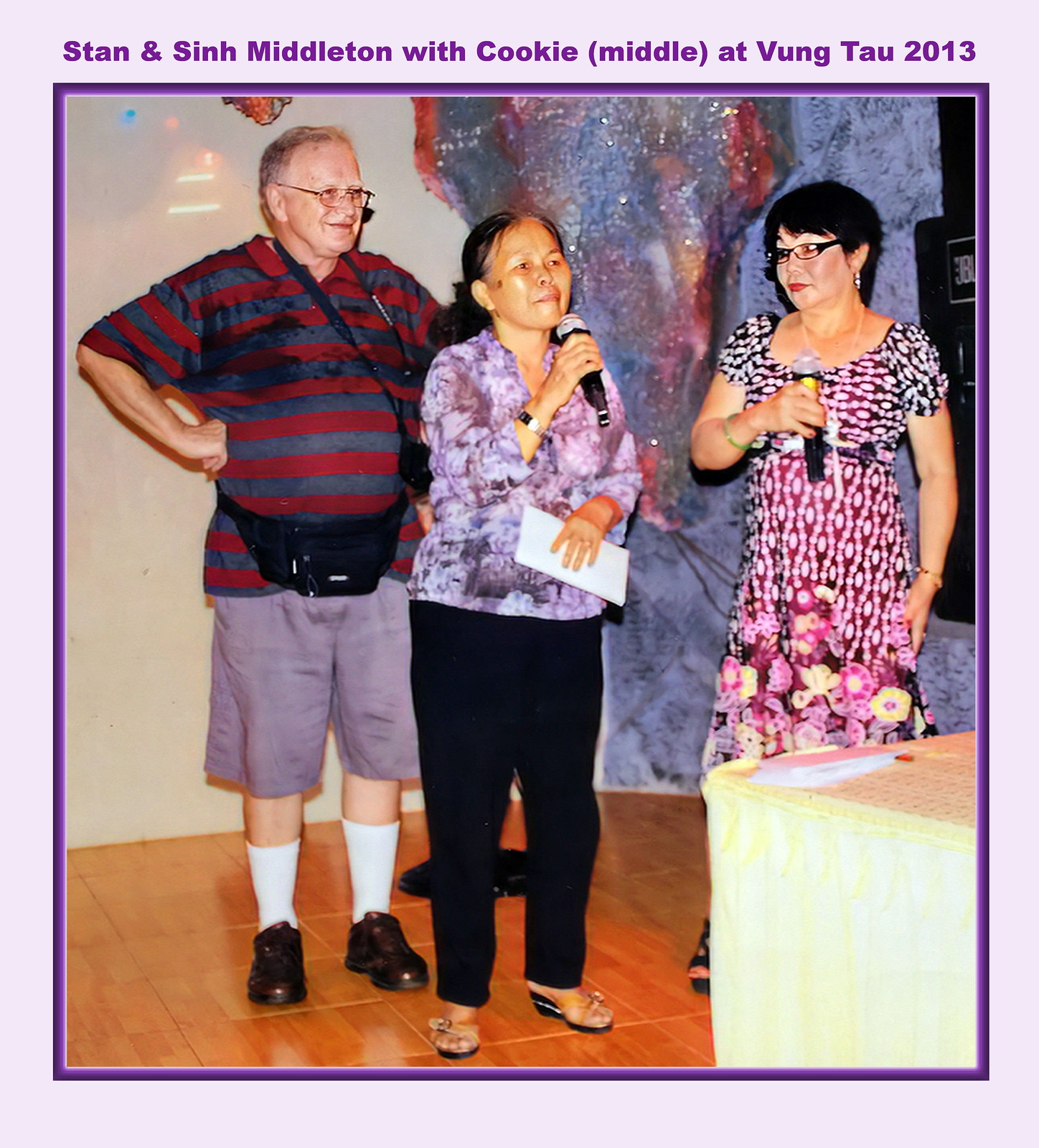This vibrant postcard image, framed with a purple border, captures a moment from Vung Tau in 2013. The scene features three individuals: an older Asian woman, a gentleman, and another woman, who appear to be engaged in a presentation or event. 

The older lady, standing confidently in a purple long-sleeve shirt and black pants with slip-on shoes, is holding an envelope in her left hand and a microphone in her right, suggesting she is speaking. To her right stands another woman, dressed in a pink floral-patterned dress, holding a microphone and looking attentively at the older lady. 

Behind the women is a gentleman dressed in gray shorts, a blue and red horizontal-striped shirt, and glasses. He wears black shoes with calf-high socks and has a fanny pack-type bag with a shoulder strap around his waist. His hands are set on his hips, and he is smiling, adding to the lively atmosphere of the scene.

The trio stands on hardwood flooring, with a background that features a mix of red and blue colors, adding depth and vibrancy to the scene. The text above the image reads, "Stan and Sid Middleton with cookie middle at Vung Tau 2013," providing context and a timestamp for this cheerful snapshot.